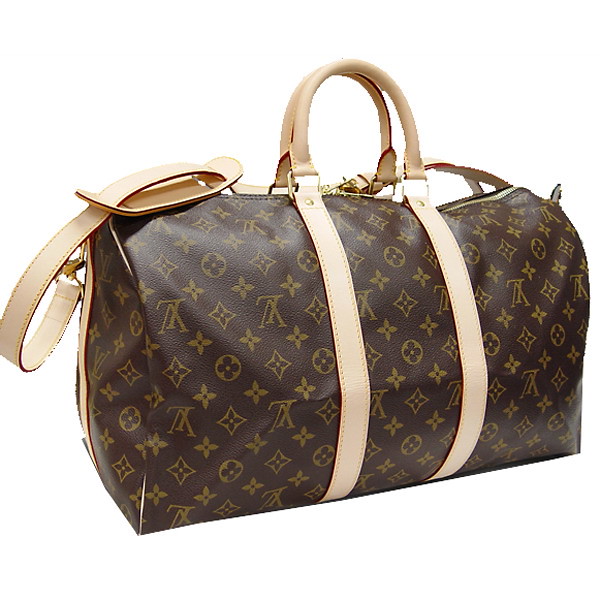This image features a Louis Vuitton handbag characterized by the brand's signature design elements. The bag is predominantly dark brown, with an oval or rectangular, small duffel bag-like shape. Its surface is adorned with the classic Louis Vuitton monogram pattern, including "LV" symbols and gold-colored, four-petaled flowers, some enclosed in circles. 

The bag is equipped with two cream-colored straps that wrap around the sides and meet at elegant, half-circle handles at the top. These handles, along with all other hardware, showcase a gold finish. Additionally, a gold zipper is visible across the top-right side of the bag. A cream-colored shoulder strap, featuring a padded section for comfort, drapes over the top and extends down the left side, looping behind the handbag. The entire scene is set against a clean, white background, emphasizing the luxurious details and craftsmanship of the Louis Vuitton piece.